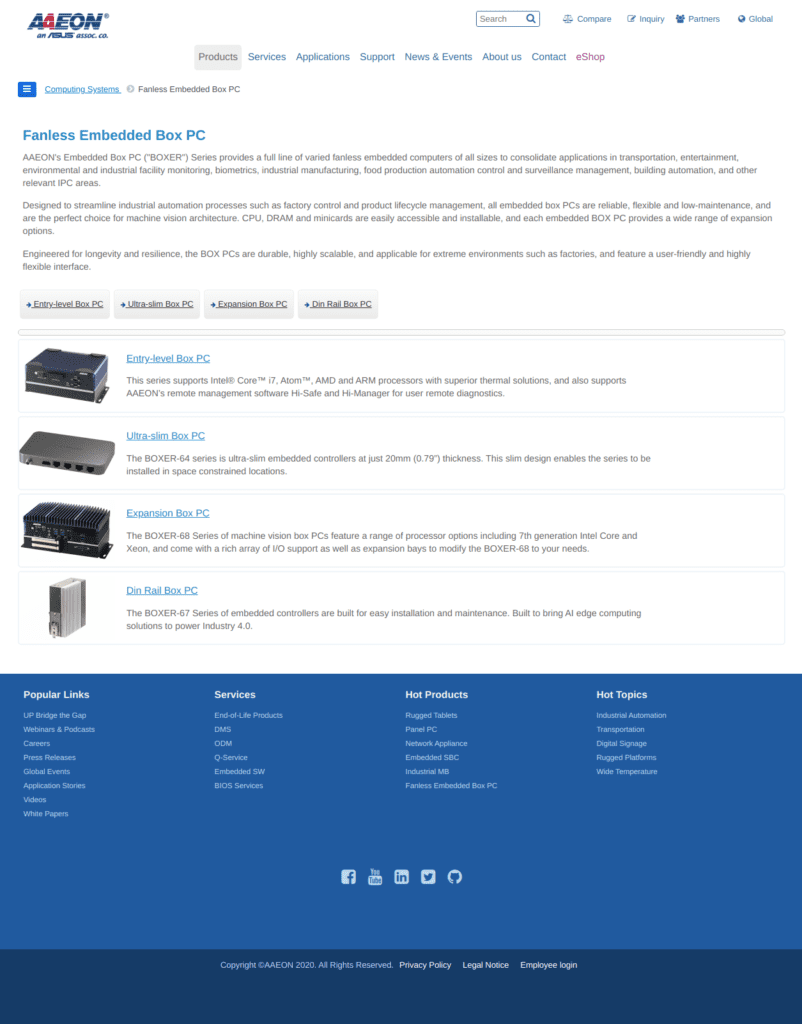Caption: 

The top left corner of the image displays the logo "Aeon," a company specializing in advanced computing solutions. Initially assumed to be related to insurance, the detailed navigation menu below reveals its focus on high-tech products and services. Options such as "Products," "Services," "Application Support," "News and Events," "About Us," "Contact," and an "eShop" indicate a comprehensive online presence. Enlarging the image further, it becomes clear that Aeon offers a range of computing systems, particularly highlighting their fanless embedded box PCs under the Boxer series. These robust, compact systems are designed for varied industrial applications including transportation, entertainment, environmental and facility monitoring, biometrics, manufacturing, food production automation, surveillance management, and building automation. The extensive detail and specific usage scenarios indicate that these products are crucial for specialized technical fields, providing essential information for prospective buyers and industry professionals.